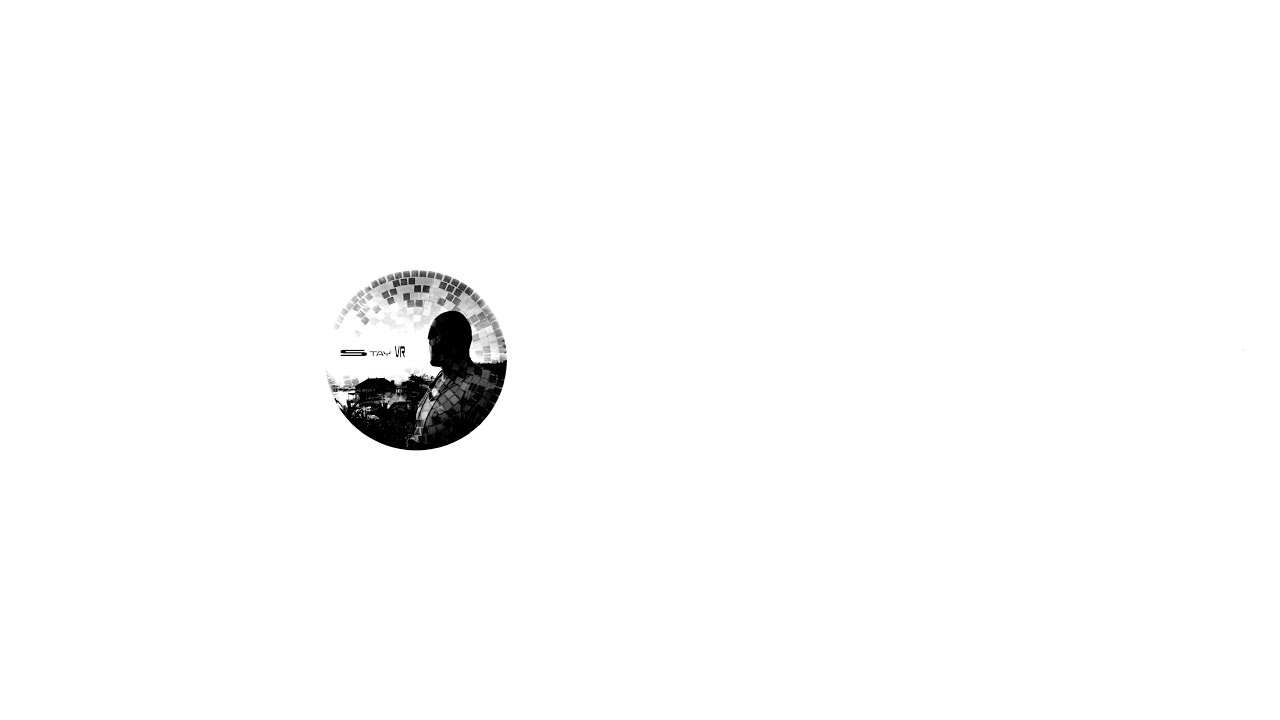The photograph is a wide black and white image dominated by a small circular inset located on the bottom left side. This circle, roughly the size of a quarter, features the silhouette of a man's head and upper chest, appearing as though he took a selfie while looking away. The man's torso is composed of dark and light gray glittery squares, reminiscent of a disco ball pattern. Surrounding the circular inset are more of these glittery squares, creating a cohesive design. In the background of this circular image, there are faint outlines of trees and buildings, possibly houses or a pier, suggesting an outdoor setting. The letters "STAY VR" are positioned vertically on the left side of the circle, adding to the logo-like composition of the image. The entire photograph maintains a monochromatic palette, with all elements in shades of black, white, and gray.